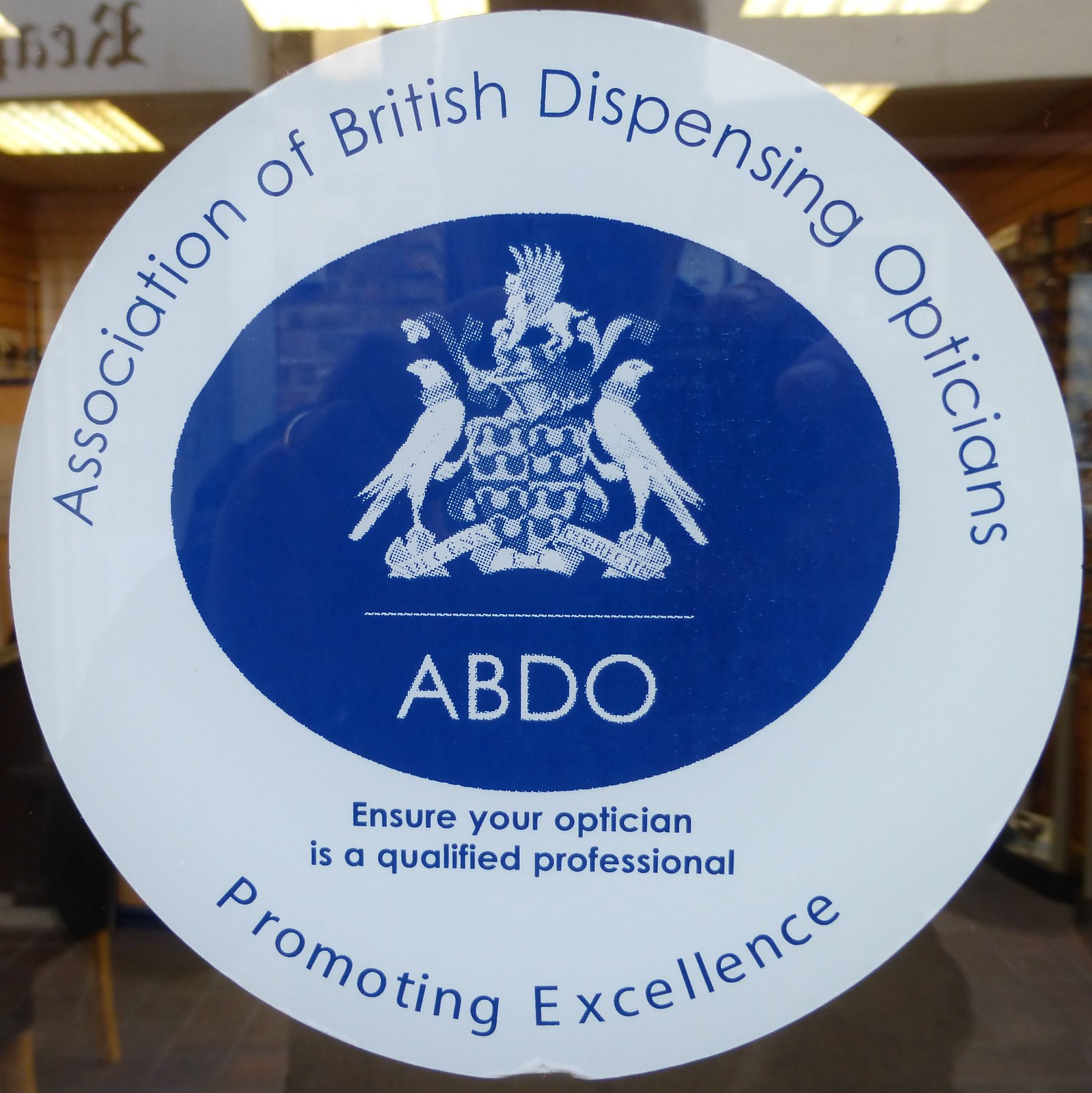This image features a blurred interior environment visible through a glass wall adorned with a prominent circular sticker. The sticker, occupying the central focus, is white with blue text and design elements. Encircling the top in an arch, the text reads "Association of British Dispensing Opticians" in blue lettering. Below this, there is a dark blue, partially transparent oval containing a detailed crest that includes birds flanking a shield, topped with a lion, and a ribbon with unreadable text at the bottom. Centrally situated within the blue oval are the bold, white, capital letters "ABDO". Further down in the white space, it states "Ensure your optician is a qualified professional," and at the bottom edge of the circle, following a curved line, it reads "Promoting Excellence" in blue letters. The background elements include fluorescent lights visibly built into the ceiling and partial legs of a chair or table visible in the bottom left-hand corner.